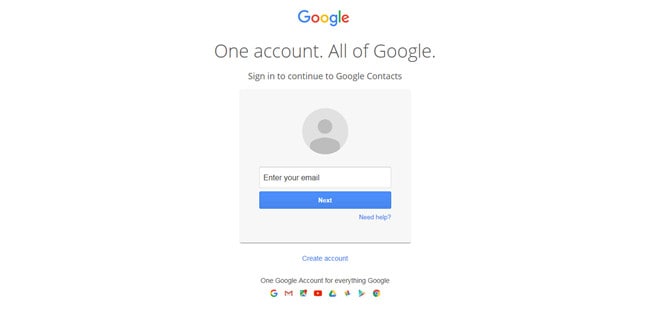The image depicts a Google account creation and sign-in page. At the top, the iconic Google logo is prominently displayed, featuring the familiar arrangement of a blue "G," a red "O," a yellow "O," a blue "G," a green "L," and a red "E," maintaining the vibrant and diverse color palette for which Google is known. Below the logo, in a large and clear font, the slogan "One account. All of Google." is visible, emphasizing the unified access provided by a single Google account.

Central to the page is a prominent gray box that serves as the sign-in interface. Within this box, there's a placeholder avatar, currently grayed out since no user is logged in. In the center of the gray box, there's a white input field prompting users to "Enter your email," inviting them to initiate the sign-in process. Beneath this input field is a blue rectangle button with the word "Next" in white text, which users press to proceed after entering their email. Additionally, a small blue link labeled "Need help?" is situated below the "Next" button, offering assistance to users who may encounter issues during the sign-in process.